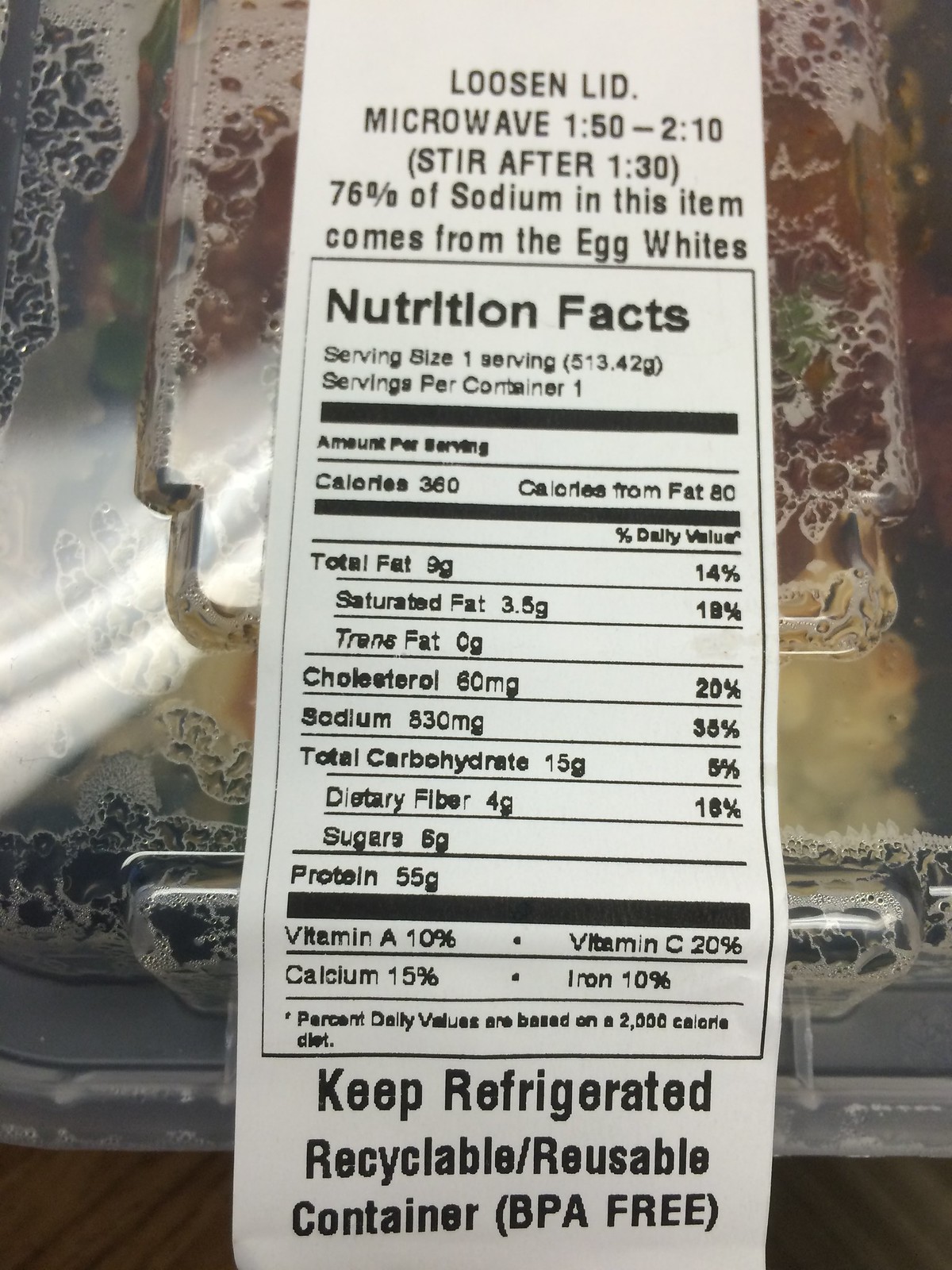A close-up photograph captures the label applied to the lid of a plastic food container, which is partially fogged with condensation, rendering the contents inside indistinguishable and out of focus. The label features detailed microwave instructions: "Loosen lid, microwave 1 minute 50 seconds to 2 minutes and 10 seconds," with a note in parentheses, "(stir after 1 minute 30 seconds)." Additionally, the label highlights nutritional information, stating that 76% of the sodium content is sourced from egg whites. It outlines further nutritional details, indicating that the single serving contained within provides 360 calories, with 80 calories derived from fat. The label elaborates on the amounts of fat, cholesterol, sodium, carbohydrates, sugars, protein, and various vitamins and minerals. At the bottom, the label instructs to "keep refrigerated" and emphasizes that the container is "recyclable/reusable" and "BPA free."